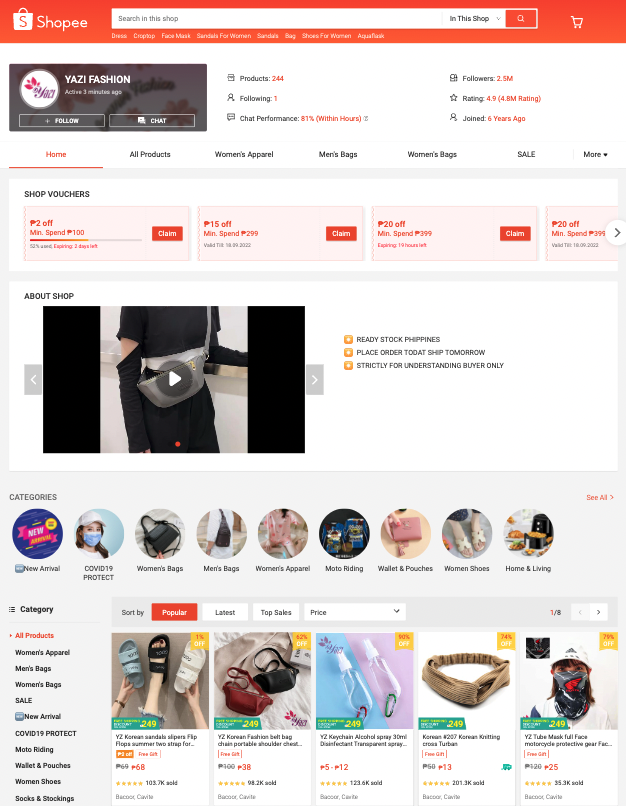### Detailed Shopping Website Screen Capture Description

**Top Section:**
The screen capture showcases a webpage from a shopping platform, identified as Shopee. At the topmost part of the image, there is an orange navigation bar featuring a white bag icon with the letter "S" on it, representing the Shopee logo. Adjacent to the logo, the brand name "Shopee" is spelled out in white text. A white search box is prominently displayed beside the logo, with placeholder text prompting users to "Search in the shop." Next to the search box, an orange and white magnifying glass icon functions as the search button. Further to the right, there is a white shopping cart icon, indicating the cart section of the website.

**Main Navigation:**
Below the top bar, though the text is somewhat blurry and small, a series of white sub-menus can be discerned. Following this section, there is an advertisement for Yazi Fashion displayed in a white section. The ad includes a round white circle with a pink butterfly icon and some text in purple font, though specific details are difficult to read due to the small font size.

**Category and Navigation Menus:**
The webpage continues with several navigation menus. An orange "Home" tab is prominently featured, followed by black text tabs for "All Products," "Women's Apparel," "Men's Bags," "Women's Bags," "Sale," and "More."

**Promotional Section:**
Below the navigation menus, there are highlighted promotions in orange boxes, offering various discounts. These include potential offers like "$2 off," "$15 off," "$20 off," and another "$20 off" voucher.

**About and Media Section:**
The "About Shop" section includes a video snapshot that appears paused. The video screen shows a person dressed in a black gown and gloves, carrying a grey bag across their chest. This section includes features such as "Ready Stock" indicated by orange boxes and three bullet points listing shop details, though the exact text is difficult to read.

**Categories and Images Section:**
Further down, there is a "Categories" section with various images:
- **New Arrivals:** Represented by a navy circle.
- **COVID-19 Protection:** Displaying an image of a woman wearing a mask.
- **Women's Bags:** Featuring a black handbag image.
- **Men's Bags:** Showcasing another black bag image.
- **Women's Apparel:** Portrayed by a pink shirt.
- **Unspecified Category:** Displayed with a black and blue circle, the exact category is hard to determine.
- **Wallets and Pouches:** Depicted with an image of a pink wallet.
- **Women's Shoes:** Illustrated by an image of a woman's feet in white sandals.
- **Home and Living:** Probably shown with an image of an air fryer.

**Footer Menus and Sorting Options:**
Further down, more category menus are visible, including "Women's Apparel," "Men's Bags," "Sale," etc., accompanied by images. The items on the site can be sorted by popularity, the latest arrivals, top deals, and price. Visible product images include sandals, purses, and other miscellaneous items.

This comprehensive and detailed caption gives a complete representation of the contents and layout of the Shopee webpage screen capture.